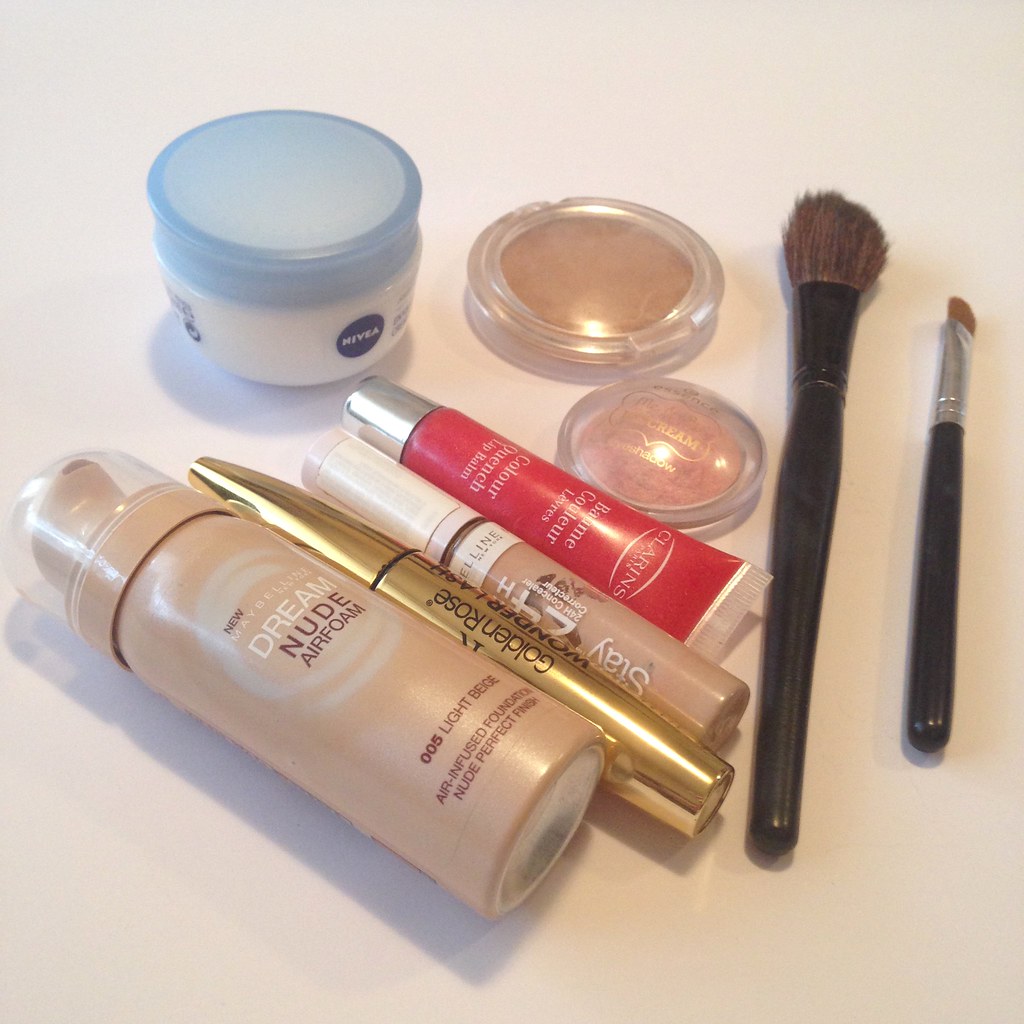A vibrant, brightly lit square photograph showcases a curated collection of skincare and makeup products against a subtle pink-tinged white background. On the right side, two vertically aligned makeup brushes with black handles are prominently displayed. The smaller brush features a large silver metal ferrule connecting the bristles to the handle, whereas the larger brush has a fluffy head, ideal for applying blush with a gentle poofing motion.

Centrally positioned are two round, flat compacts. The larger compact contains a brownish foundation or blush, while the smaller one has a reddish-pinkish hue. Diagonally crossing the scene is a red squeeze tube of Clarins Color Quench Lip Balm, identifiable by its silver screw-on lid.

Adjacent to it is a Maybelline Stay 24 Hour Foundation, with a twist-off lid likely revealing an applicator. Another item close by is a golden tube of Golden Rose Wonder Lash, assumed to be mascara. Nearby, a canister of Maybelline Dream Nude Air Foam in shade 005 Light Beige stands out, featuring an air-pumped dispenser with a clear acrylic cover.

In the top left corner sits a classic Nivea jar, made from white glass with a blue screw-on lid, likely containing cold cream. The meticulously arranged assortment of products is bathed in overhead light, highlighting their varied textures and colors.